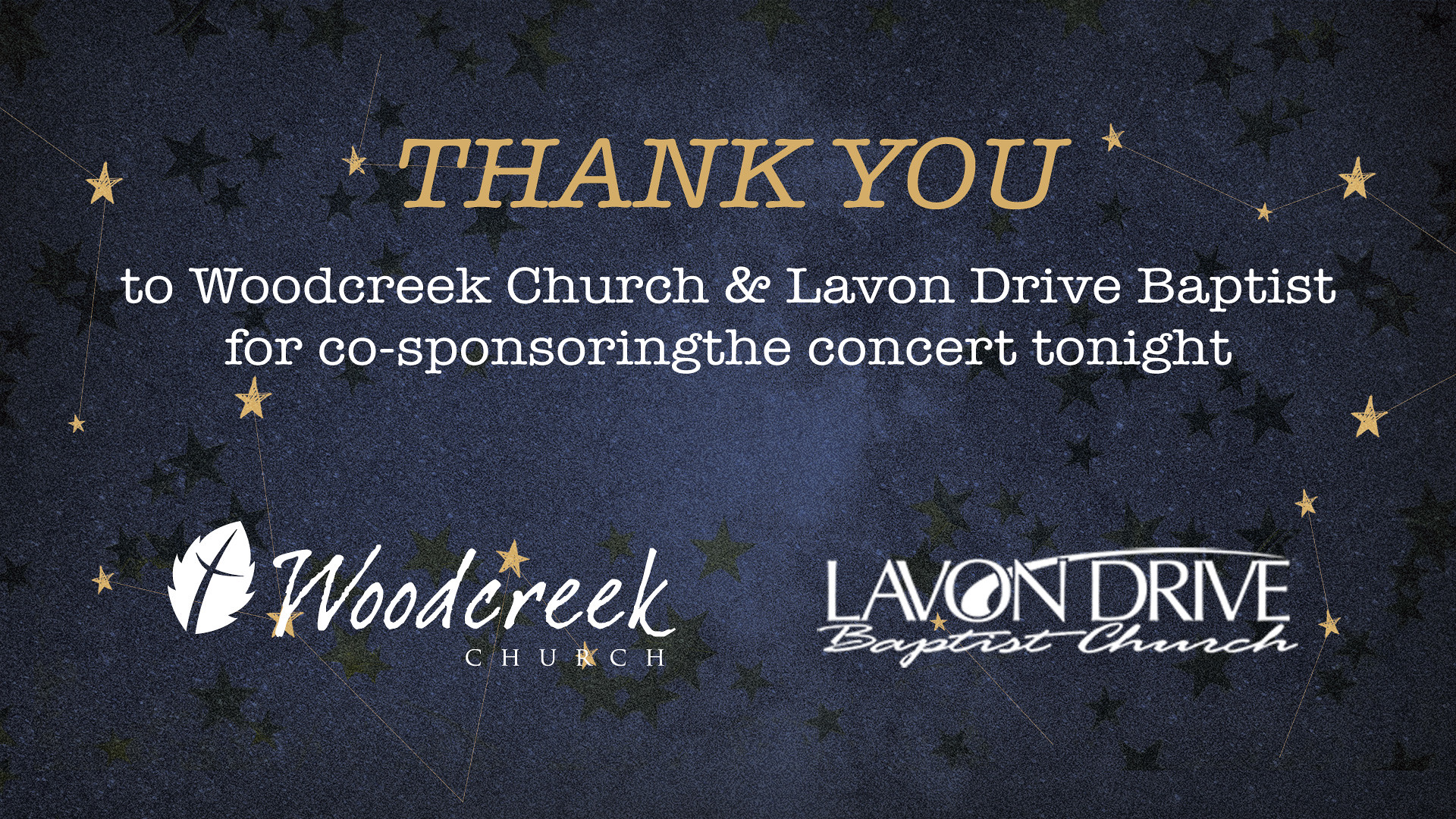The image depicts a digital thank-you card with a background that resembles a dark night sky, adorned with black and golden star shapes. The center of the background is slightly lighter, transitioning to a darker hue around the edges. 

At the top, centered, is the phrase "THANK YOU," written in bold, golden letters. Below this, also centered, are two rows of white text in a basic Times New Roman font that reads, "to Wood Creek Church & Lavon Drive Baptist for co-sponsoring the concert tonight."

The word "and" is replaced by an ampersand, and there is no space between "co-sponsoring" and "the."

At the bottom left of the card is the logo for Wood Creek Church, which includes an image of a leaf. On the bottom right is the logo for Lavon Drive Baptist Church. Both logos are in white. The overall size of the image is comparable to a business card, maintaining a compact and professional appearance.